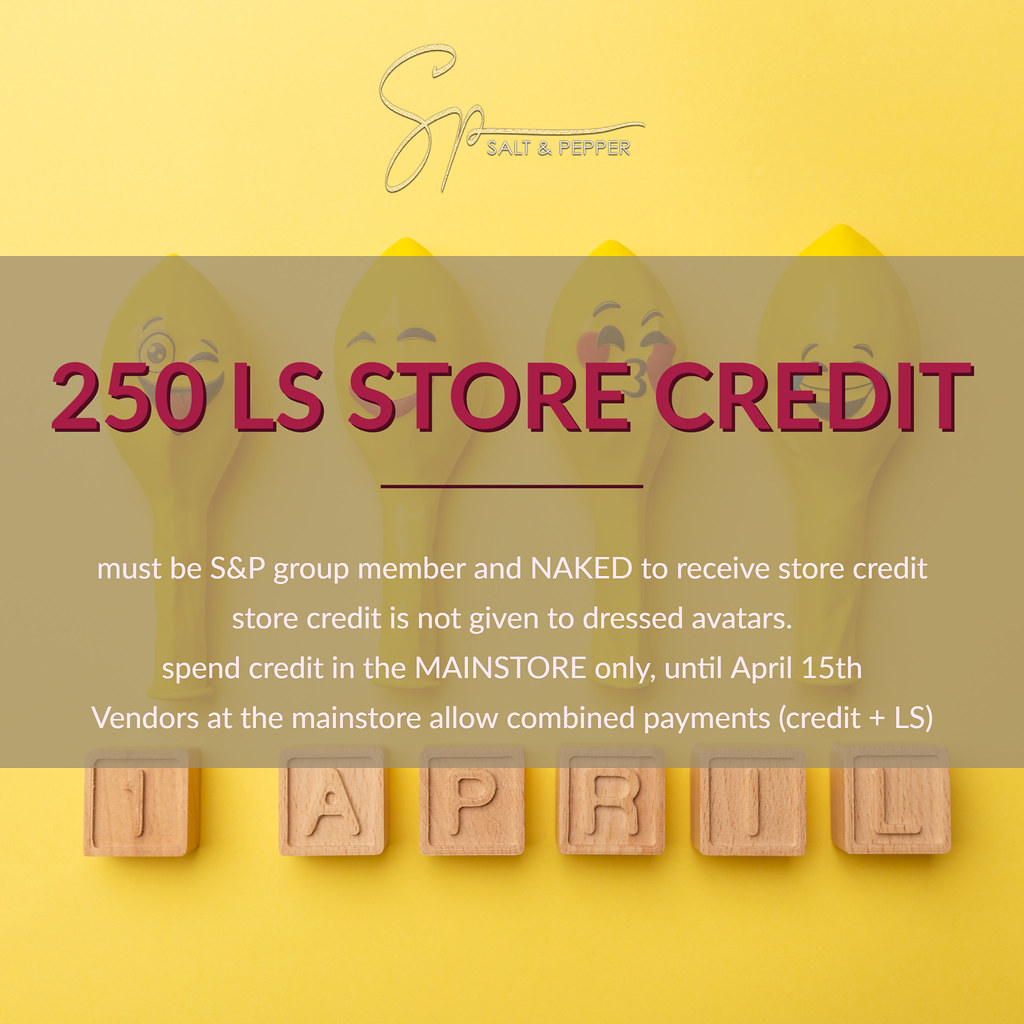The square advertisement features a predominantly yellow background with four spoons, each displaying a different face, resembling deflated balloons. At the top of the image, a logo reads "Salt-N-Pepa" or "SP" in a cursive style. Centered in bold red text is the announcement "250 LS Store Credit." Below this, additional white text states that to receive the store credit, one must be a Salt-N-Pepa group member and naked, as store credit is not given to dressed avatars. The credit is valid in the main store only until April 15th, and it notes that vendors at the main store allow combined credit plus LS payments. At the bottom, wooden blocks spell out "1st April," hinting at a possible April Fool's promotion.